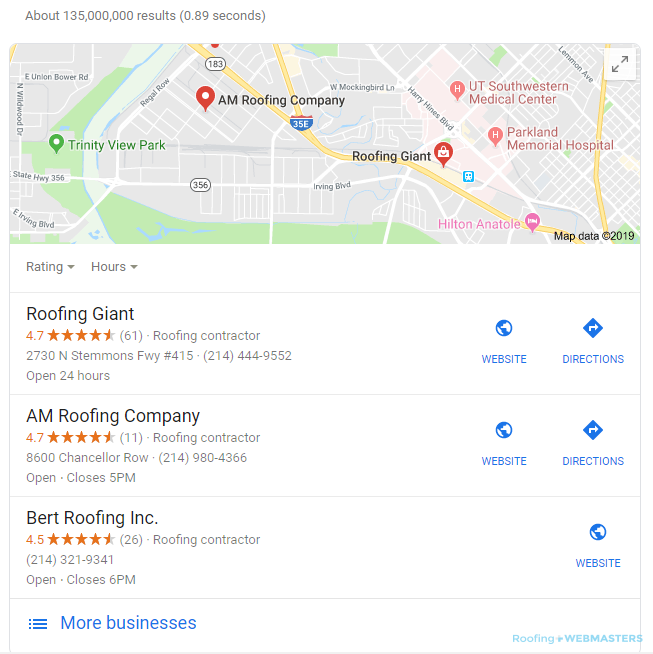This screenshot from Google Maps showcases search results for roofing companies in the vicinity of Trinity View Park. At the top, the page indicates there are approximately 135 million results generated in 0.89 seconds. 

The map section highlights the locations of AM Roofing Company and Roofing Giant, both situated near UT Southwestern Medical Center and Parkland Memorial Hospital. 

Below the map, there are filters for "Rating" and "Hours." Following this, three businesses are listed:
1. **Roofing Giant**: Boasts a 4.7-star rating based on 61 reviews, with options for a website and directions.
2. **AM Roofing Company**: Also has a 4.7-star rating but from 11 reviews, featuring options for a website and directions.
3. **Burt Roofing Inc**: Holds a 4.5-star rating from 26 reviews, offering a website but no direction link.

At the bottom, there’s a link to view “More businesses.” On the right side of each business row, the logo "Roofing+ Webmasters" is present.